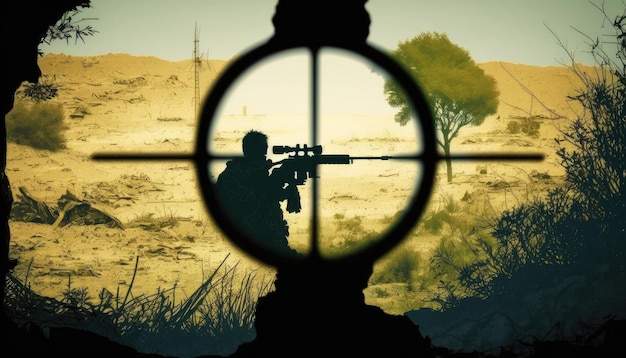The image depicts a war scene set in a desert landscape, featuring a light brown to golden terrain with the ridge of a hill near the top of the frame and a yellowish-blue sky overhead. Dominating the barren landscape is a tree with a skinny brown trunk and branches topped by a yellowish-green canopy, standing out against the desolate backdrop. Adding depth, the image has a bluish-black silhouette of grass and bushes framing it, with the silhouette extending into an overhanging rock at the top left corner. 

The central focus of the scene is through the scope of a sniper rifle, identifiable by the distinctive black circular viewfinder with a crosshair aimed at another sniper rifle. This second rifle, also black, points to the right and is held by a silhouetted figure to its left. The environment surrounding this intense focal point shows some scrub brushes and what appears to be dark foliage. In the distance, near the hill, a pole with wires—or potentially a radio tower—adds to the desolate, battle-scarred atmosphere. The vignette effect around the edges of the image enhances the dramatic and immersive nature of this war zone depiction.